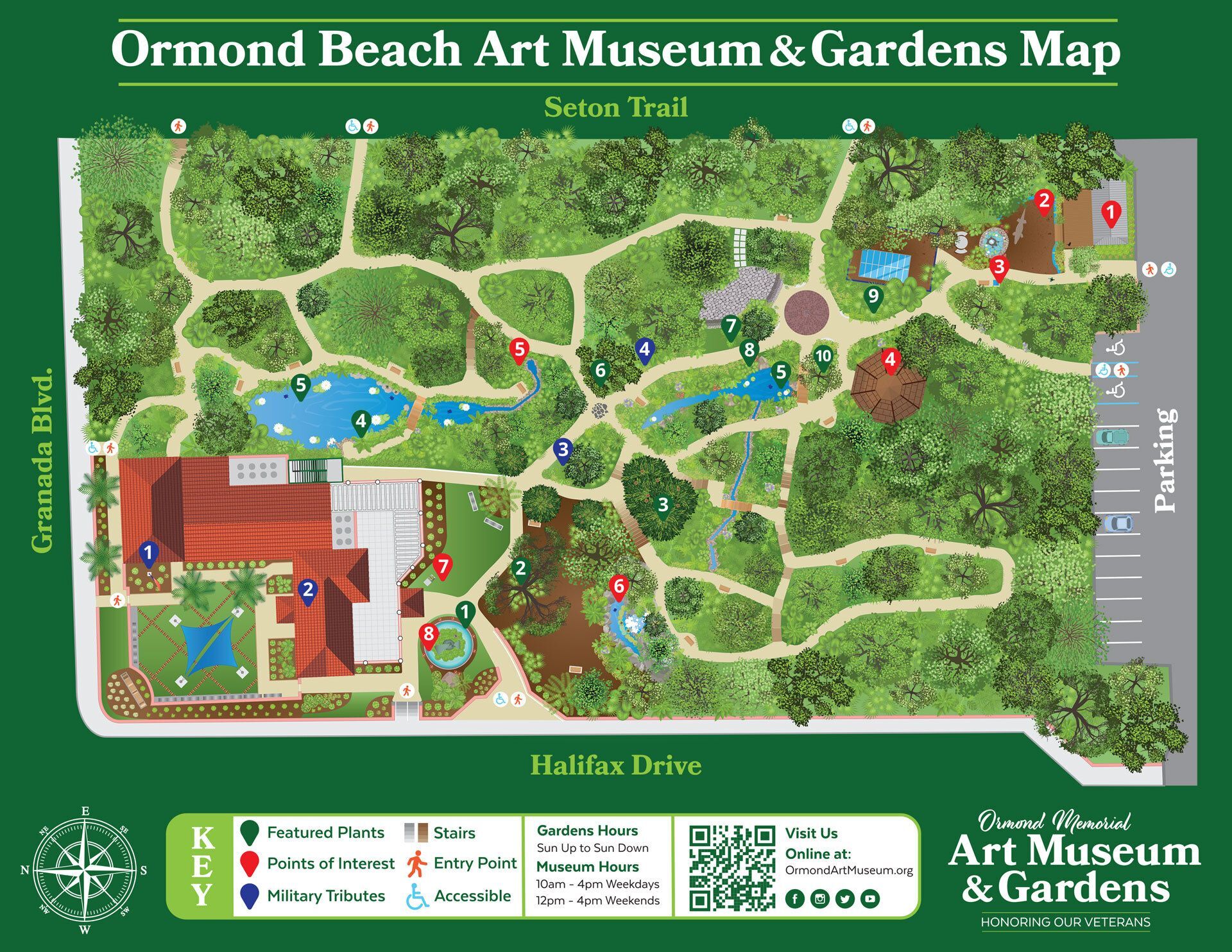The image depicts an intricately detailed map of the Ormond Beach Art Museum and Gardens. The entire map is set against a green background, with the title "Ormond Beach Art Museum and Gardens Map" prominently displayed in white at the very top. The map features a 3D aerial view of the facility, highlighting the Seton Trail with numerous trees and pathways in light tan color. Various colored circles denote different locations and features, with a key provided at the bottom explaining their meanings: green for Featured Plants, red for Points of Interest, blue for Military Tributes, gray and blue for Stairs, orange for Entry Points, and blue for Accessible areas. Important landmarks such as Granada Boulevard on the left and Halifax Drive at the bottom guide visitors through the map. Additionally, a large building complex is visible, alongside parking areas, and a separate text in the bottom right states "Ormond Memorial Art Museum and Gardens Honoring Our Veterans." A compass located at the bottom left aids in orientation, completing the comprehensive layout of this visitor guide.